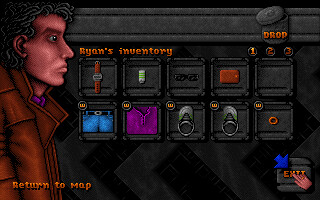This is a detailed screenshot from an older video game, likely from the 1990s. On the left side of the image, there's a computer-generated character - a Caucasian man with medium-length brown hair, black eyes, and a neutral, slightly serious expression. He's dressed in a tan leather jacket over a purple shirt. The man is visible from just above his waist up and is facing to the right.

In the center of the screen, there's a grid labeled "Ryan's Inventory" in a bronze-colored font. The inventory consists of five slots wide and two slots tall, with various items including a watch, sunglasses, a phone, a tube of something, sneakers, shorts, a shirt, a ring, and a wallet. 

The top right corner of the screen has a small trash can icon labeled "Drop," suggesting the option to discard items. Below this are three tabs, with the first tab currently selected. In the lower left corner, there's a button labeled "Return to Map," and in the lower right corner, there's an "Exit" button with a hand cursor and a blue arrow pointing to it, indicating that you can leave the screen.

Overall, the image showcases a character beside an inventory management screen typical of video games from the late 20th century.